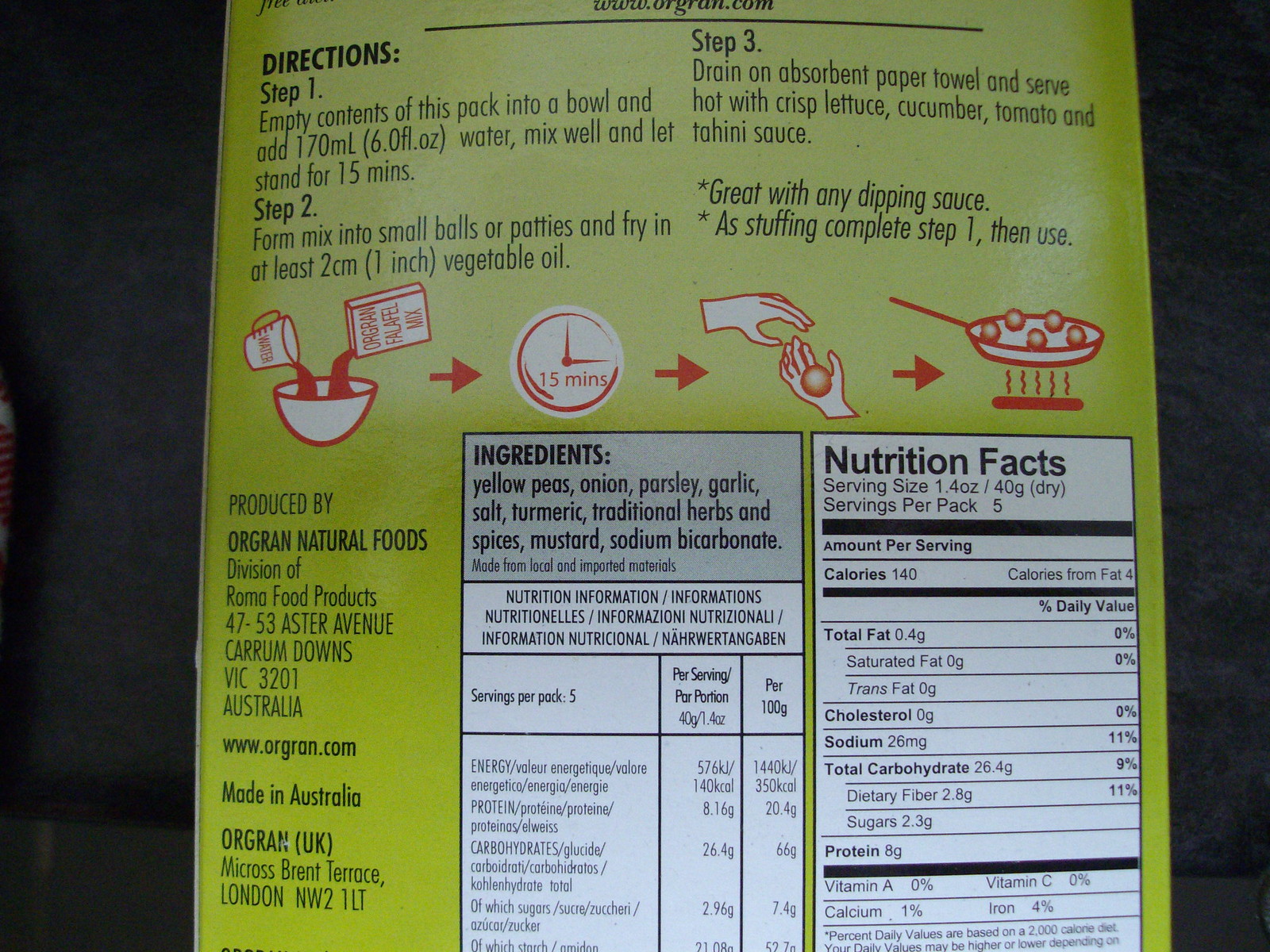The image depicts the backside of a food package predominantly colored in shades of green. Detailed instructions for preparing the packaged food are outlined in three distinct steps, each accompanied by red and white illustrations visually guiding through the preparation process. To the left of the instructions, the package prominently displays the producer's name, website, and the manufacturing location. The lower section provides a comprehensive list of ingredients and a nutritional facts panel, which is set against a white background and bordered in black. This panel meticulously details essential dietary information including serving size, calories, fat content, carbohydrates, and protein.